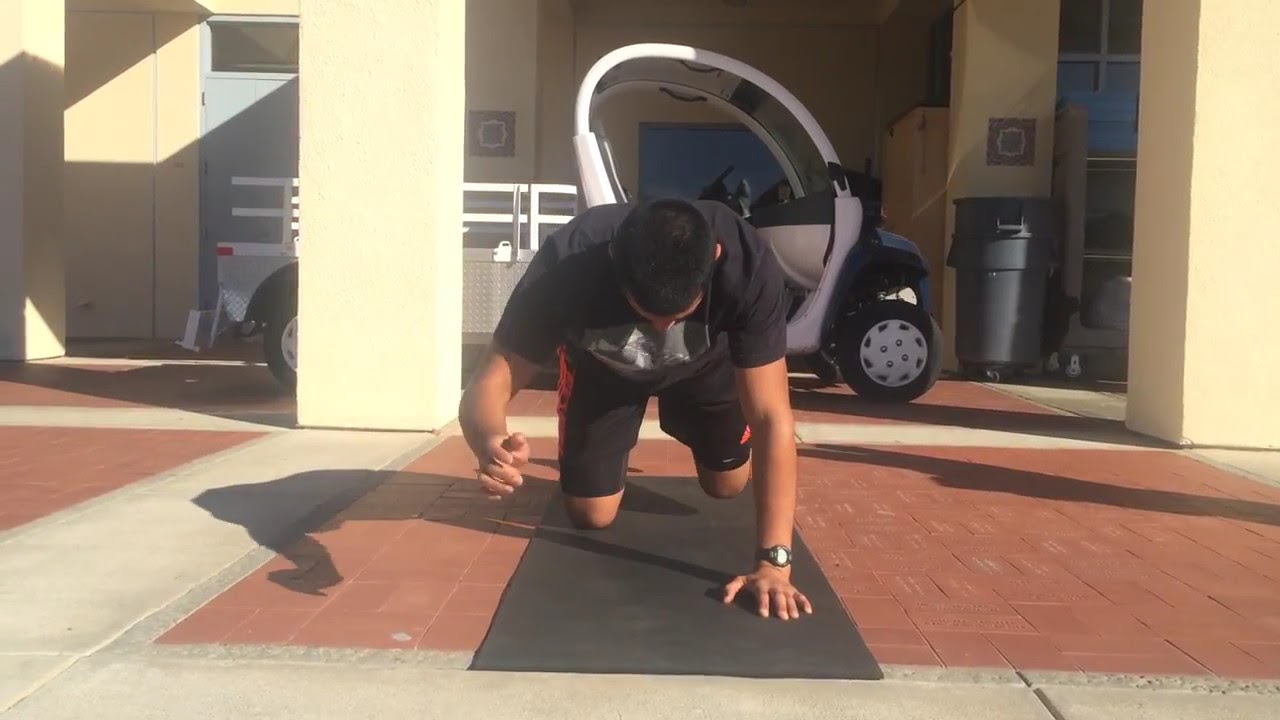This outdoor photograph captures a man engaged in a yoga pose on a grey mat, placed on a red brick-paved area, possibly in a courtyard of a public or business building. The man, with short black hair, is positioned on his hands and knees, appearing to be in a modified push-up position. His right hand and left knee are elevated, while his left hand and right knee are grounded on the mat. He is wearing a black t-shirt and black and red shorts, with a watch visible on his wrist. The strong sunlight casts a clear shadow of him to his left, as well as another indistinct shadow suggesting the presence of another person off-camera. In the background, there's a white vehicle resembling a golf cart or utility cart parked near a large grey-black trash can on wheels. The building behind them features cream-colored walls and a blue door, as well as beige pillars that add to the architectural detail.